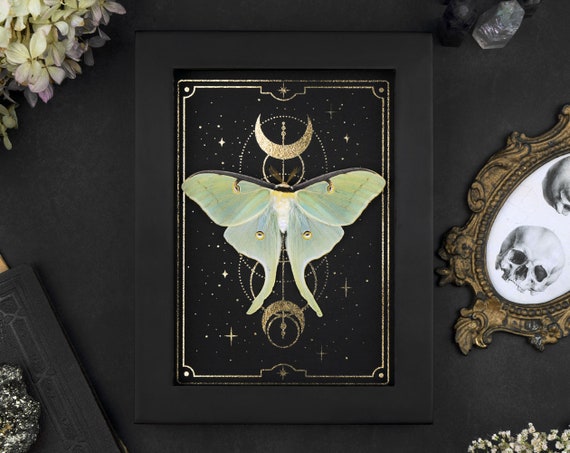The image features a charcoal gray background with a detailed composition. In the upper left-hand corner, a portion of a white flower with delicate, tiny blossoms is visible. The lower left corner similarly showcases small white blossoms, while additional white blossoms appear in the lower right corner. 

Centrally placed is a decorative gold frame with an ornate design, featuring a white oval center. Within this center, a skull is depicted at the bottom portion and a partial skull is visible at the top portion. Overlaying this, there is what appears to be a white crystal knob with a black metal attachment.

In the middle of this complex scene, another frame appears—charcoal gray with gold edges. Inside this frame lies a white and green butterfly, with its body colored white and wings displaying a very pale green adorned with gold markings. Above the butterfly, gold markings form a moon, a crown, and a half circle, adding a celestial touch. Below the butterfly, a moon facing the opposite direction and several circles contribute to the intricate, layered design.